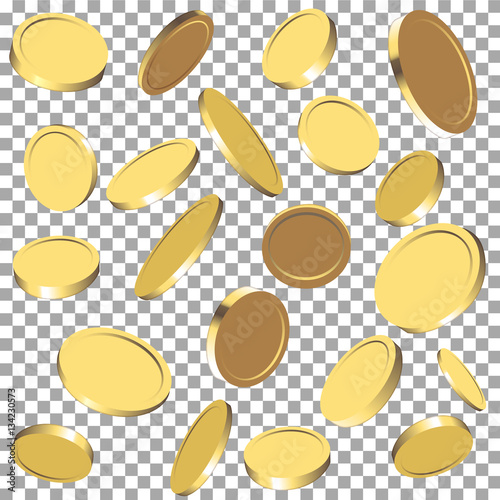The image features numerous gold coins scattered across the frame in various orientations, displaying different angles of the same object. Some coins appear shinier and lighter due to the glare, while others, facing away from the light, exhibit darker, brownish hues. The background consists of a small, even checkerboard pattern in white and gray, suggesting an intended transparent background for web use. The coins are evenly distributed throughout the image without overlapping. The only visible text on the screen reads "Adobe Stuck." The overall color scheme includes shades of gold, white, gray, and a hint of black, giving the image a polished and reflective digital appearance.